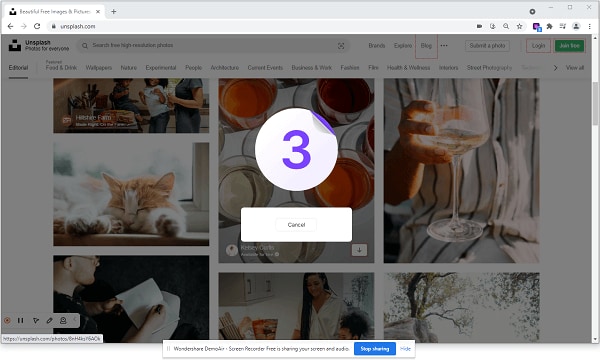The image depicts a screenshot of a web browser interface. At the top left corner, there's an open tab, followed by a back button and a refresh button. To the right of these buttons is a search field for entering website URLs. On the far right, there's a cluster of small icons that are not clearly discernible due to their size.

The main focus of the screen is a grayed-out website overlaid by a white circle in the center displaying the number "3" in purple. Directly below this circle, there's a prominent "Cancel" button. Additionally, it appears that the screen is currently being shared, as indicated by a long rectangular bar at the bottom of the screen featuring a "Stop Sharing" button.

In the background, the website appears to host a collection of photographs. Among these images, one features a person holding a wine glass, and another shows a cat sleeping by a window, suggesting a variety of different photos.